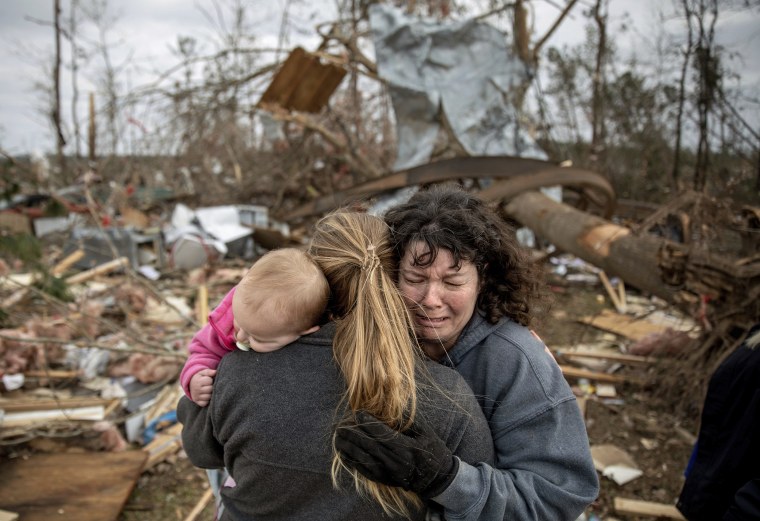In this poignant photograph taken during daylight, three women stand in the foreground amidst the heartbreaking aftermath of a natural disaster, likely a tornado. The older woman with curly brown hair and wearing a blue hoodie and black gloves is visibly distraught, her eyes filled with tears as she embraces a younger woman. The younger woman, with long honey-blonde hair, faces away from the camera and holds an infant dressed in a pink jacket against her shoulder, a gesture of protection and comfort. Surrounding them is a landscape of devastation: a large tree lies knocked over, possibly having crashed into a house, and the ground is littered with debris—including pieces of wood, fabric, and other remnants of personal belongings—highlighting the storm's fury. The sky above is a grim gray, adding to the somber mood of the scene. The dominant colors in the photograph are brown, pink, gray, with occasional spots of blue and green peeking through the wreckage, painting a vivid picture of the calamity's aftermath.